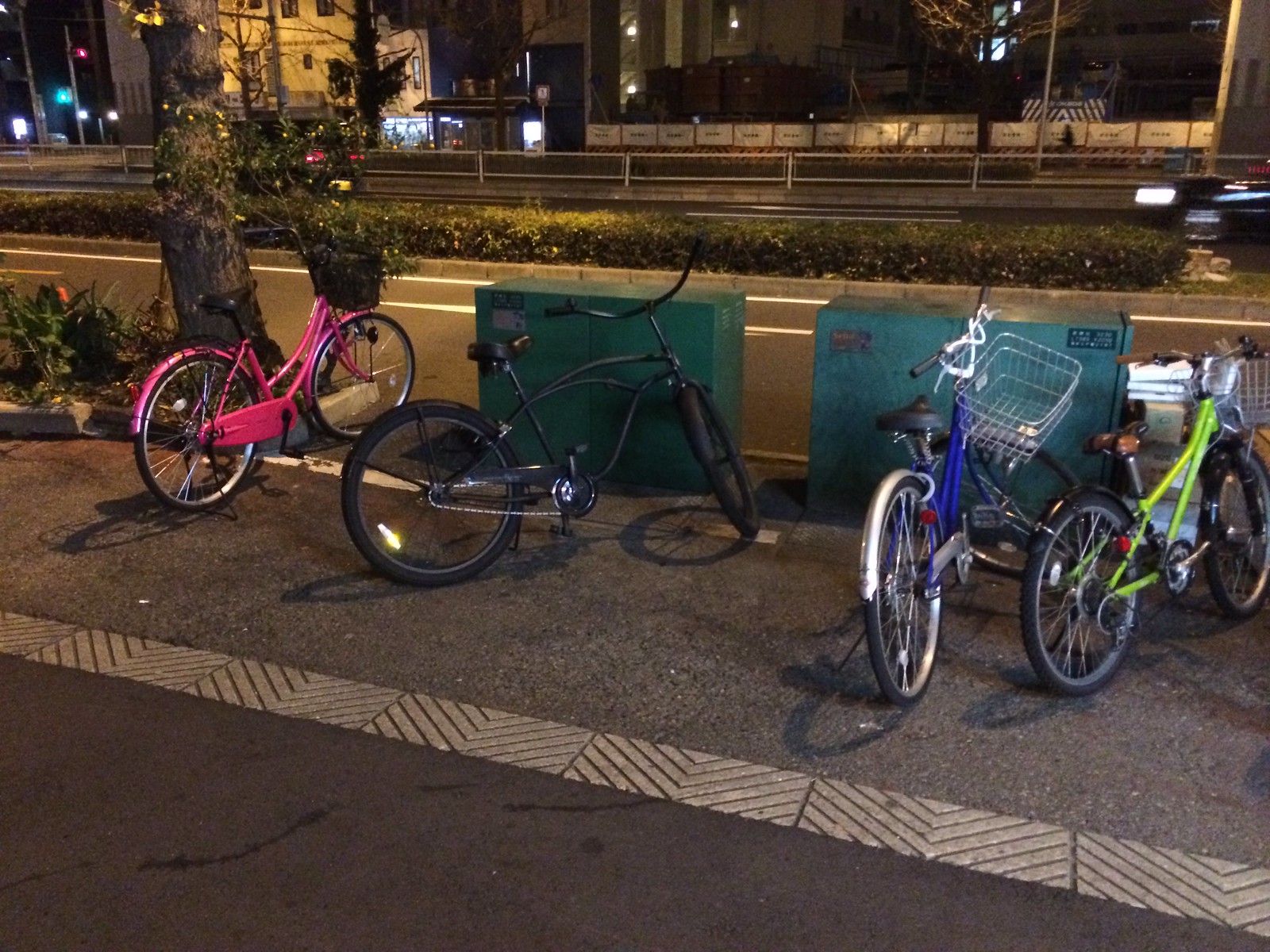This is a nighttime photograph taken on a city street, depicting four bicycles parked along a gray and black pavement sidewalk near a roadway. To the left of the scene, a tree trunk is visible. Positioned in front of the bikes are two large green electrical transformer-style boxes. The bikes are arranged from left to right: a bright pink women's style bike with a black seat and no basket, a black bike with an all-black frame and a rear reflector but no basket, a navy blue women's bike with black handlebars, a black seat, a silver fender, and a silver basket, and a neon green women's bike with a silver basket and a black seat. The sidewalk is separated from the roadway by a median with bushes. In the background, there are silhouettes of traffic lights, a bus stop, some buildings with lights still on, and a construction zone, indicating a bustling urban setting.